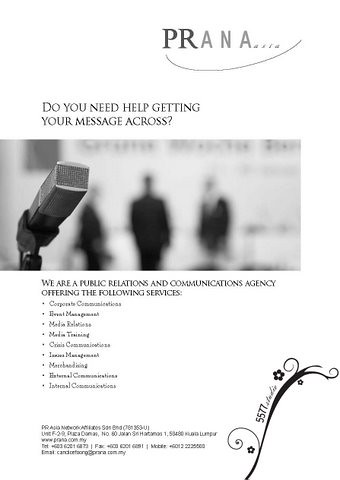The advertisement for Prana prominently features a black-and-white image of a square-shaped microphone in focus, while three blurred figures stand in the background, creating a narrow depth of field. At the top left, the Prana logo is displayed, with "PR" in bold and "ANA" in smaller gray letters followed by a swoosh. The headline of the ad reads, "Do you need help getting your message across?" indicating the core offering of the company. Below the microphone image, a text block states, "We are a public relations and communication agency offering the following services." A bulleted list follows, though most items are difficult to read due to pixelation and blur. Visible services include media relations, media training, corporate communications, internal communications, and crisis communications. At the bottom, there's contact information, including phone numbers, addresses, and an email, which is challenging to decipher. To the bottom right, an additional logo with a flowery emblem and the numbers "5577," possibly indicating their address or studio name, is featured in a cursive style that's hard to read. The entire advertisement is set on a white backdrop and presented in grayscale.